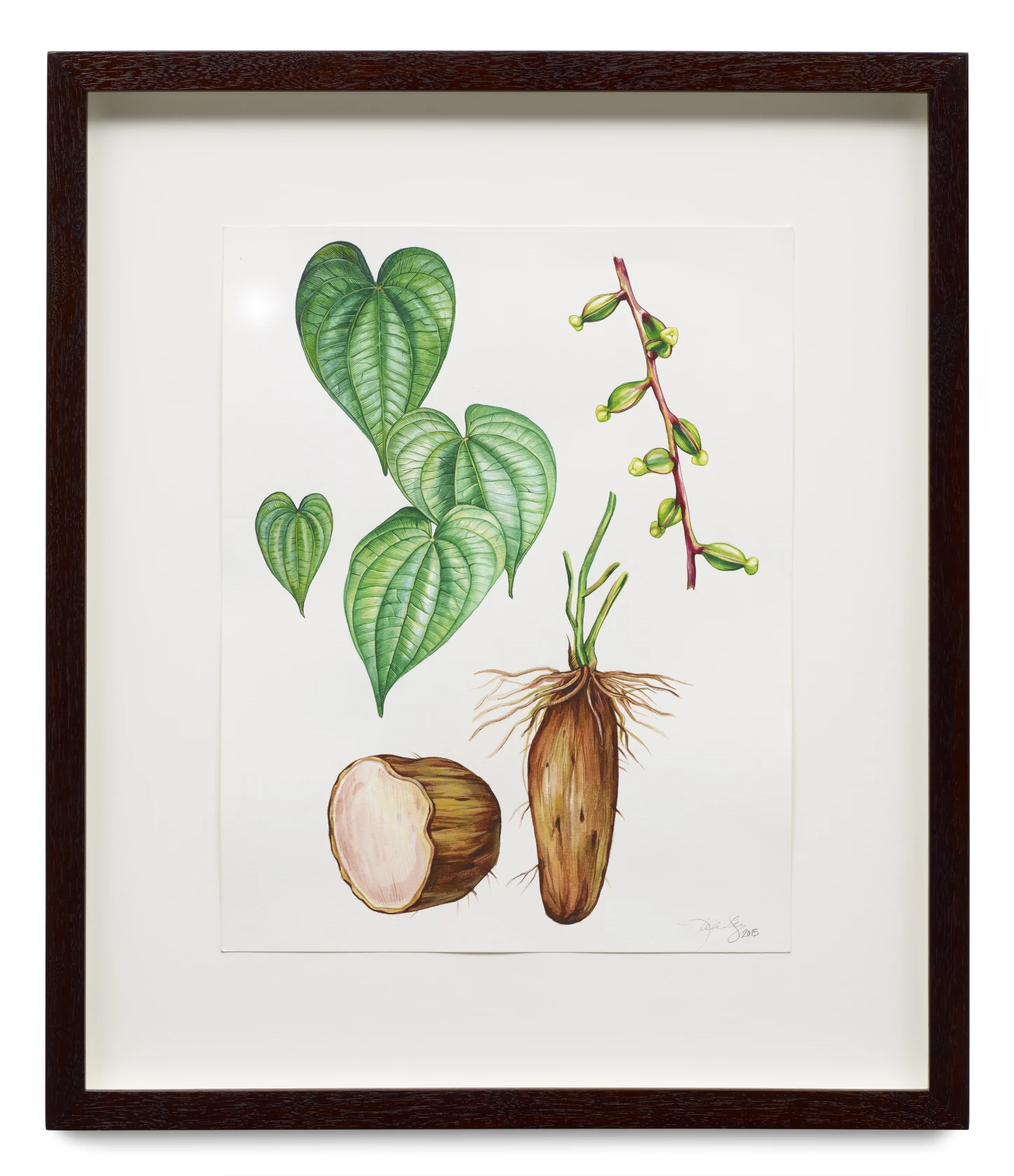This photograph captures a framed piece of artwork, elegantly enclosed in a dark wood frame with a pristine white background. The centerpiece is a colorful drawing meticulously crafted on a white sheet of paper. The drawing features heart-shaped green leaves, each vein and contour clearly defined, growing from a slender stem adorned with green buds. Below, the composition includes a detailed illustration of a root system: a large root or vegetable attached to the stem, depicted with roots splaying outwards. Adjacent to this, there’s a detailed cross-section of the same root or vegetable, revealing its intricate internal structure. The framing and detailed artwork together create a visually compelling piece that combines elements of botanical illustration and artistic expression.